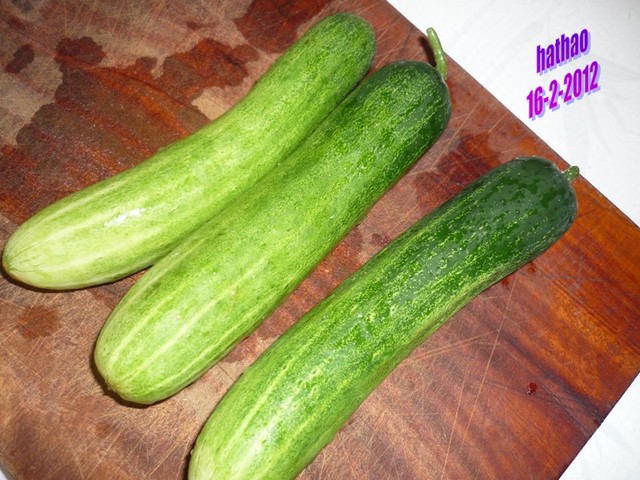This photograph captures three medium-sized, green vegetables likely to be cucumbers, though they could also be zucchinis. Each vegetable exhibits a gradient from light green at the bottom to darker green at the top, with one of them retaining its stem. They are placed side-by-side on a well-worn, reddish-brown wooden cutting board that bears multiple knife marks, indicating frequent use. The cutting board is still damp, suggesting that the vegetables were recently washed. To the right of the cutting board, a white background features the text "hathao" written in lowercase purple letters, followed by the date "16-2-2012."